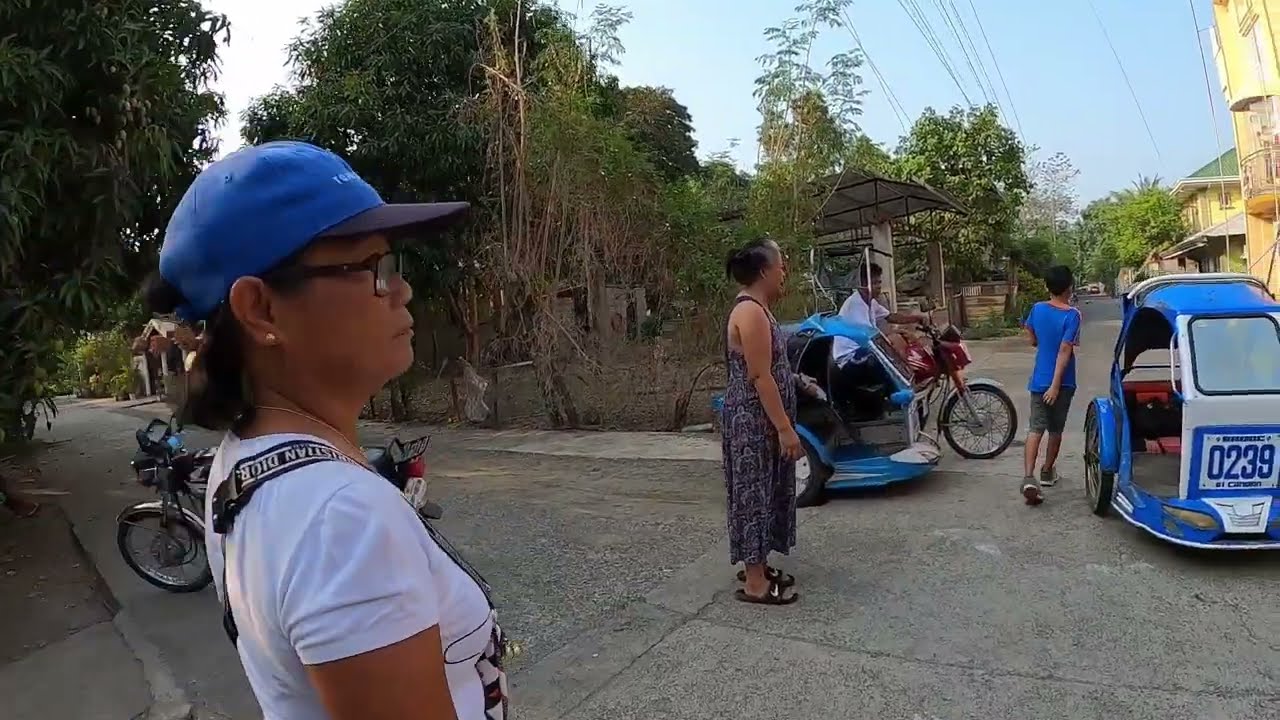In this detailed image of a bustling street scene, we observe a stone sidewalk stretching along the right side and bottom edge of the frame. The sky and trees with some power lines are visible at the top. At the center of the image stands a gathering of people and various small vehicles. Notably, a man is seated on a red motorcycle with a white shirt, positioned next to a child in a blue shirt and brown pants. An older woman in a floral dress and sandals stands nearby, alongside another woman with a blue ball cap, white shirt, and glasses, who has a camera strapped across her shoulders.

Two blue, cart-like vehicles, adorned with the number '0239,' can be seen parked near the sidewalk, appearing as if they function as passenger carts or taxis. The stone sidewalk, marking a significant part of the scene, extends leftwards, interspersing the gathering. Behind the vehicles and people, a stone fence and green trees are noticeable, reinforcing the outdoor, daytime setting that hints at an Asian country. The vivid colors in the image range from light blue and white to green, brown, tan, purple, gray, and silver, painting a lively and diverse street tableau.